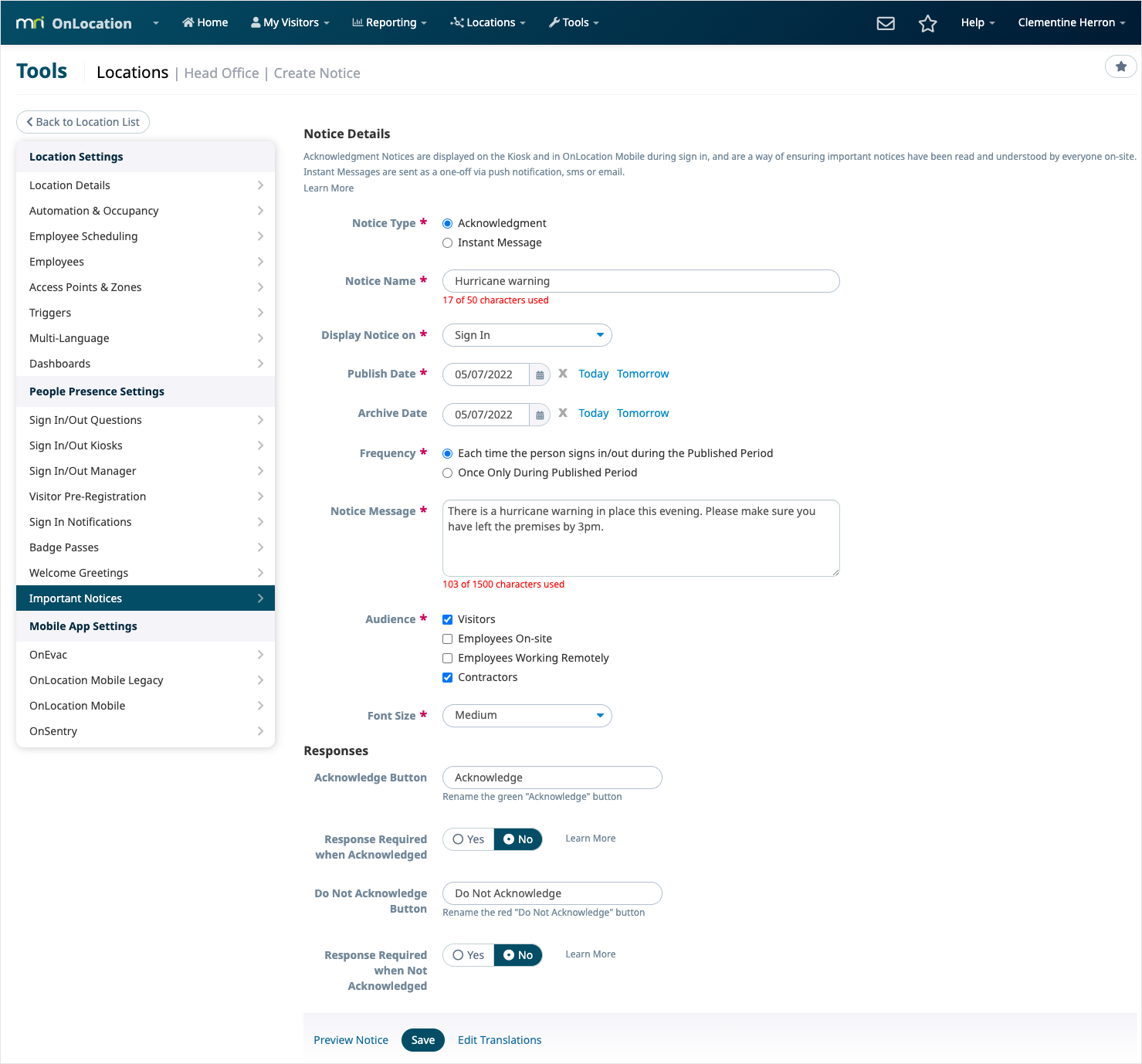A screenshot of a website interface is shown, featuring a dark blue-greenish menu bar that spans across the top. On the upper left-hand side of the menu bar, the text "MRI on Location" is prominently displayed, indicating the website's branding. To the right of this, there are several menu options laid out in a row. These include "Home," "My Visitors," "Reporting," "Locations," and "Tools." Further to the right, the menu bar includes icons for different functions: a mail envelope icon for messages, a star icon which presumably serves as a favorites shortcut, a help dropdown menu, and lastly, the user profile displaying the name "Clementine Heron" with a dropdown for additional user options.

Beneath the menu bar, the screen is divided into sections. On the left, written in a greenish-blue font, the word "Tools" is visible. To the immediate right of this, "Locations" is displayed in black font. Further to the right and in gray font are "Head Office" and "Create Notice," with a small star button at the far end of this line.

Directly below this area, an array of panes is present, beginning with a "Back to Location List" button on the left-hand side. Underneath, the "Location Settings" section is visible, featuring eight selectable options. Following this, there's a "People Present Settings" section containing seven different adjustable options. An important notices banner is also evident, followed by a "Mobile App Settings" section that includes four options.

On the right-hand side, occupying the main portion of the screen, are the "Notice Details" and "Responses" sections. Each of these sections contains several fields for user input, allowing for detailed customization and response collection.